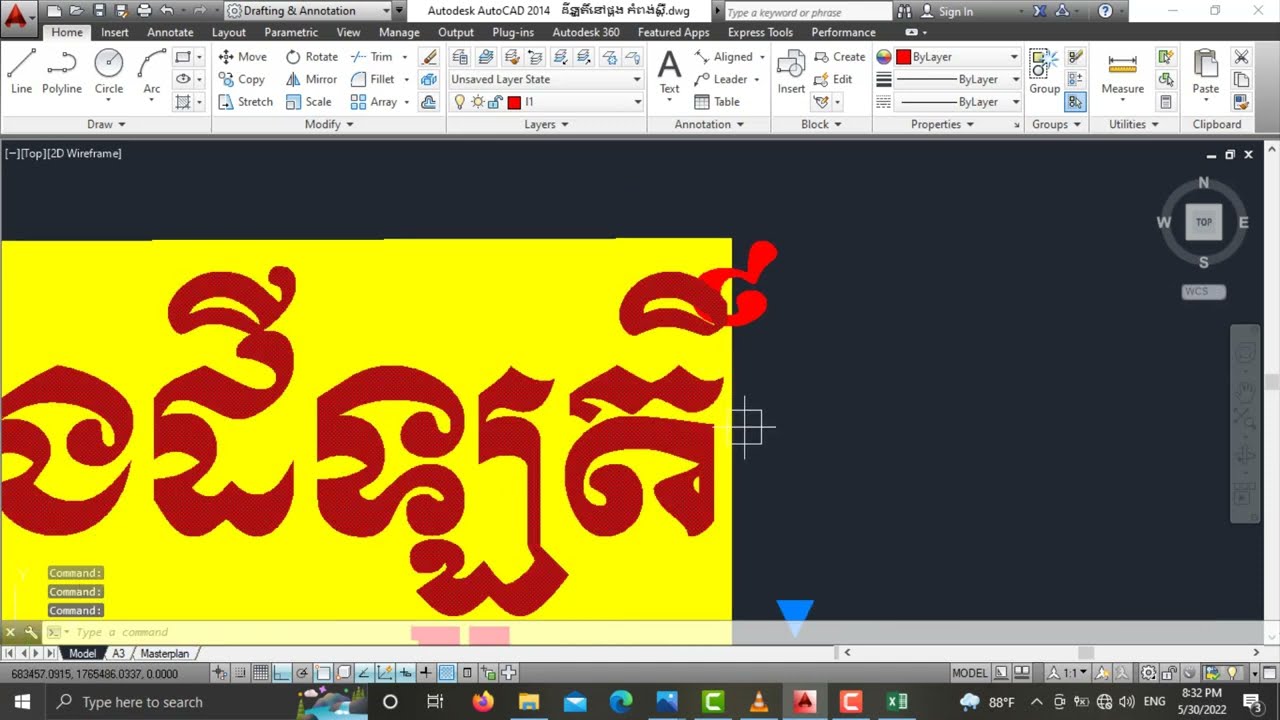The screenshot depicts a detailed view of a Windows interface with a drafting or design application, possibly Autodesk AutoCAD 2014, open in the center. The desktop layout includes the standard Windows taskbar at the bottom. On the left side of the taskbar, there is the Windows Start menu icon and a search bar labeled "type here to search." Adjacent to these are several application icons, such as Firefox, File Explorer, email, and Microsoft Edge, along with other utilities. On the right side of the taskbar, typical system icons are visible, showing weather at 88 degrees and rainy, battery status, speaker volume, time and date, and notifications. 

The design application interface itself features several English-labeled tabs such as Home, Insert, Annotate, Layout, View, Manage, Output, Plugins, Autodisc 360, Featured Apps, Express Tools, and Performance. There's a prominent dark gray header and footer, with various drawing tools like line thickness, textures, and color options displayed at the top. The workspace has a dark blue-gray background. Within this workspace, a gold rectangle with red text, which appears to be in Middle Eastern or Arabic script, is positioned towards the left, possibly indicating a foreign design aspect. Other design elements include a compass with directional markers North, West, East, and South, implying the drafting of a project that may require orientation. The overall setting of the application window is bright and clear.